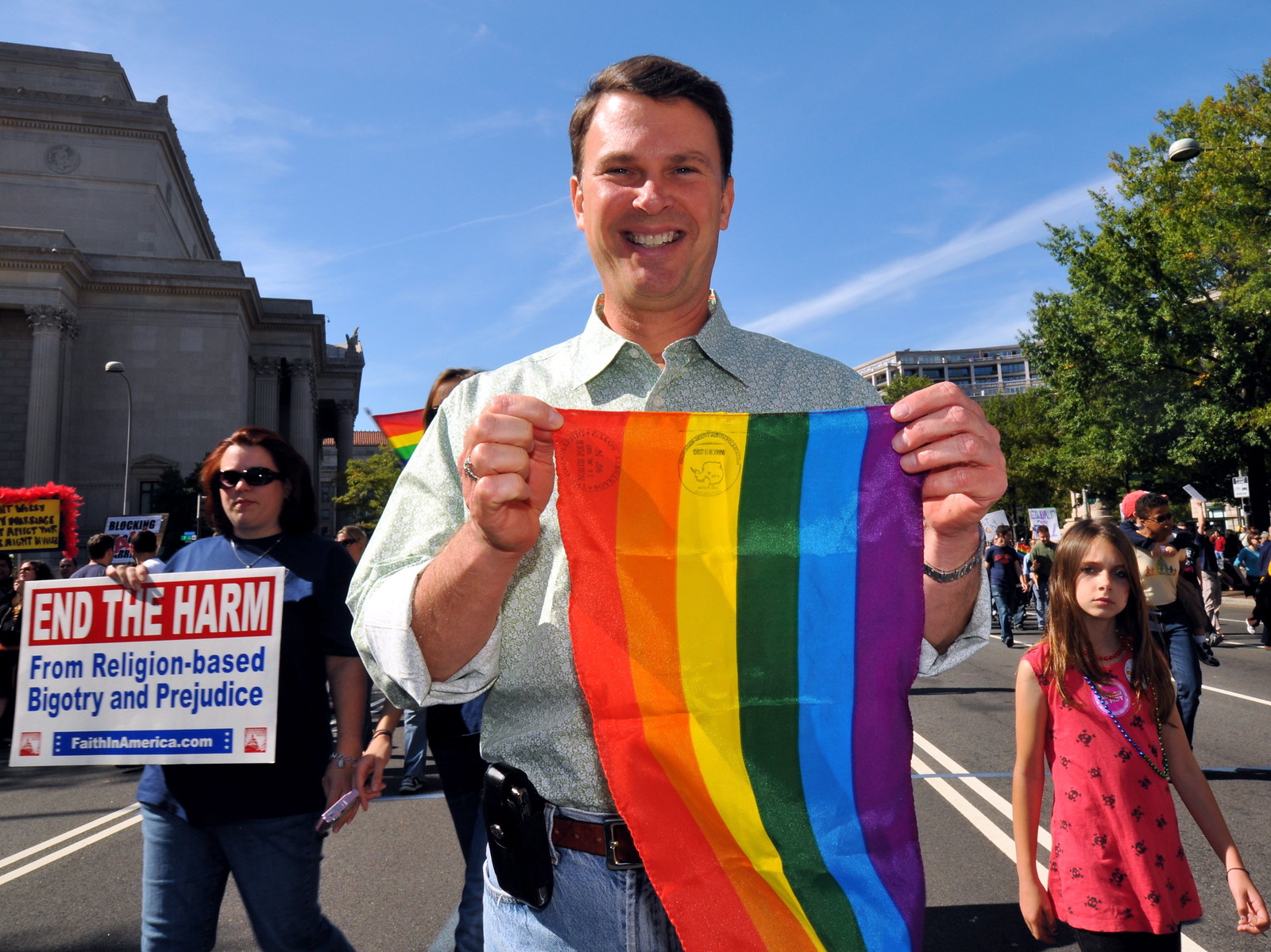In the image, a lively pride parade unfolds on a clear, sunny day. Central to the scene is a man, aged around 30 to 35, smiling broadly at the camera. He has short brown hair and is clad in a greenish-white button-up shirt with sleeves rolled up, and blue jeans. The man proudly holds a vertically positioned, vibrant rainbow banner featuring the colors red, orange, yellow, green, blue, and purple. To his right is a young girl with dark brown hair cascading over her ears. She is wearing a red blouse adorned with brown stars and a strap over her right shoulder. Adjacent to the man on his left, a woman in a dark blue t-shirt and blue jeans is also a notable figure. She wears sunglasses and holds a sign with a red, blue, and white design that reads "End the Harm" in red at the top. Below, in white, it says, "From Religious-Based Bigotry and Prejudice," and further down in blue, it references "FaithInAmerica.com." The background is bustling with numerous marchers, some holding signs and rainbow flags. A young girl walking alongside him looks up at the camera, while behind them is a man carrying a child piggyback. On the left side of the image, there's a stately granite library building with grand columns, while to the right, an office building can be faintly seen. Upper right, a large tree spreads its branches over the road, enhancing the urban environment with its lush greenery. The sky above is a perfect blue, dotted with a few puffy white clouds, capturing the parade's vibrant and inclusive spirit.